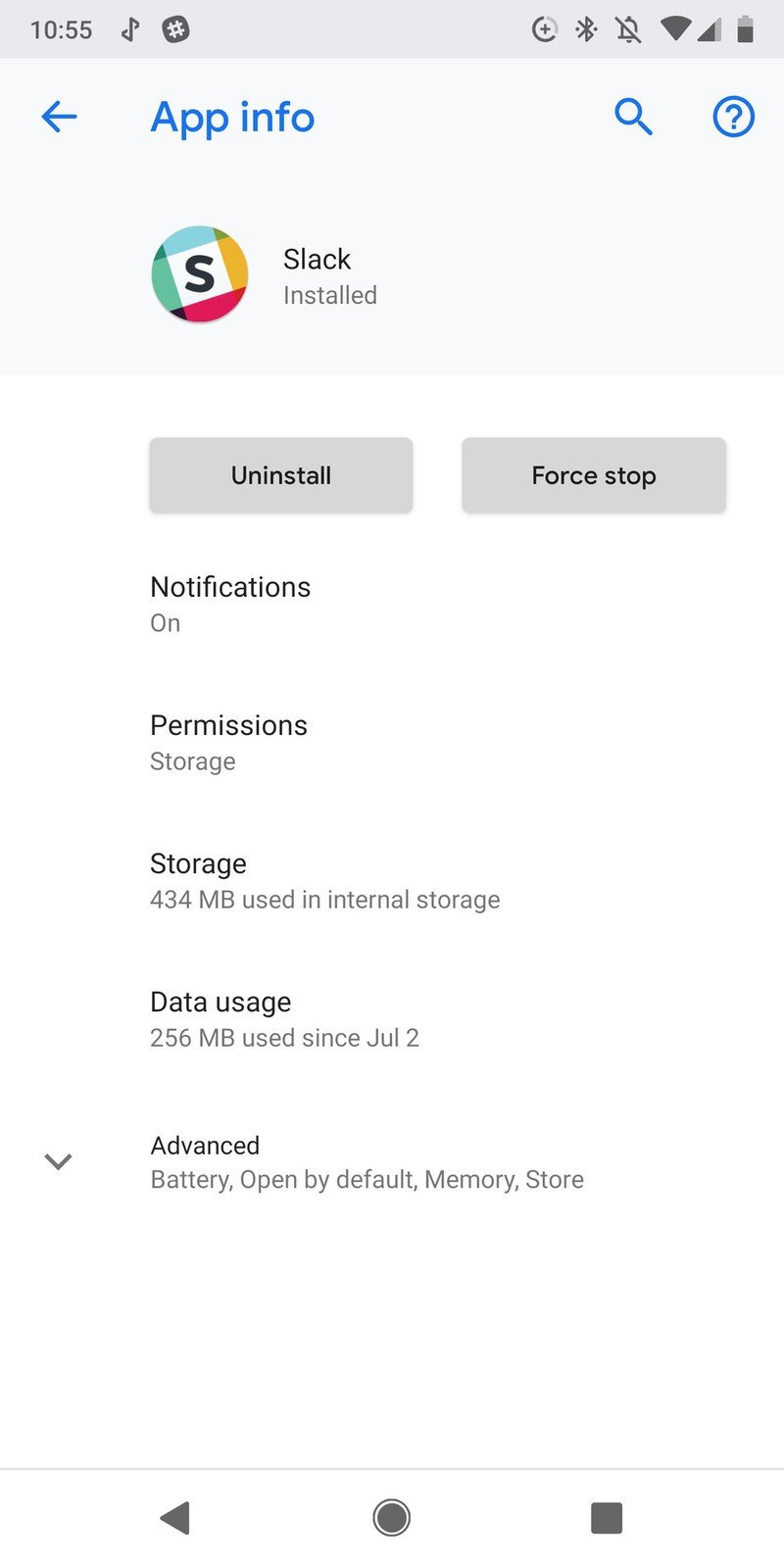A detailed screen capture of a smartphone interface is displayed, showing the system time as 10:55 AM and the battery level at approximately 75% charged. The screen is labeled "App Info," indicating that the user is exploring application details. The app in focus is "Slack," and its status is marked as "installed."

Several options are visible: users can choose to either "Uninstall" or "Force Stop" the app. Notifications for Slack are enabled, and multiple sections provide further details: "Permissions," "Storage," "Data Usage," and "Advanced settings." Under the "Storage" section, it's noted that Slack consumes 434 MB of internal storage. The "Data Usage" section reports that 256 MB of data has been used by Slack since July 2nd.

If "Advanced settings" is selected, additional information such as battery usage, open-by-default settings, and memory usage specifics will be available. At the bottom of the screen capture, there are three control buttons: a "rewind" button, a "stop" button, and a "record" button, likely indicating that this screen capture was taken during a screen recording session.